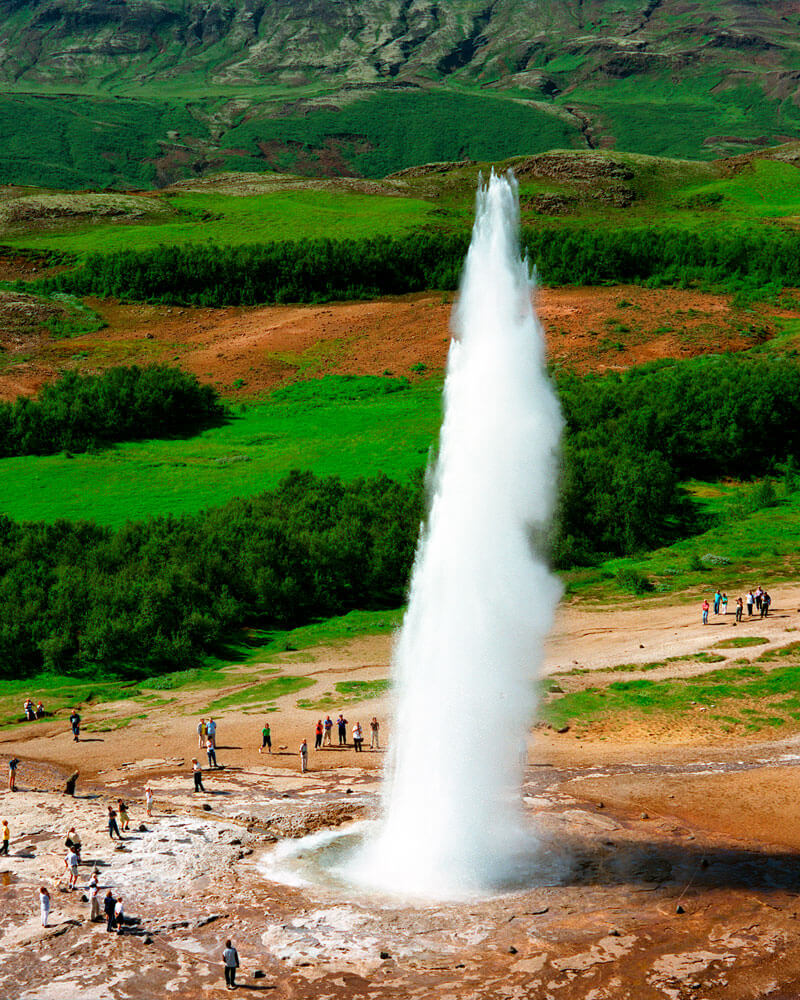In this captivating image, a towering geyser erupts dramatically, shooting high into the air, surrounded by a landscape of stunning natural beauty. In the background, majestic grayish mountains with green vegetation provide a breathtaking backdrop. Rolling hills with green grasses stretch out in front of these mountains, gradually giving way to a series of smaller, grassy mounds and interspersed dirt patches. Curving into the foreground, a scattering of trees outlines the scene, leading towards a dirt and grassy area.

At the forefront, the geyser dominates, drawing the attention of numerous onlookers who have gathered in a semicircle to witness its powerful display. These spectators, many with cameras in hand, are capturing the spectacle from various vantage points, with the majority clustered in the lower left corner of the image. Their expressions suggest awe and excitement, adding a lively human element to this natural wonder.